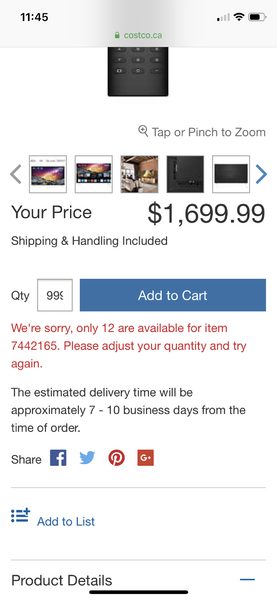The image displays a screenshot from a Costco.ca product page. At the top of the page, the time is shown as 11:45. Beneath the time, there is a prompt reading "Tap or pinch to zoom." In the URL box, "Costco.ca" is visible. The price of the item is listed prominently as "$1,699.99," with a note that shipping and handling are included. 

The quantity selected is "0.99", alongside a blue "Add to Cart" button. Below this, in red text, a warning states, "We're sorry, only 12 are available for item 7442165. Please adjust your quantity and try again." The estimated delivery time is noted as approximately 7 to 10 business days from the time of order.

Further down, social media share buttons for Facebook, Twitter, Pinterest, and Google Plus are displayed. Below a dividing line, there is a blue hyperlink that reads "Add to List," followed by another dividing line and a section titled "Product Details."